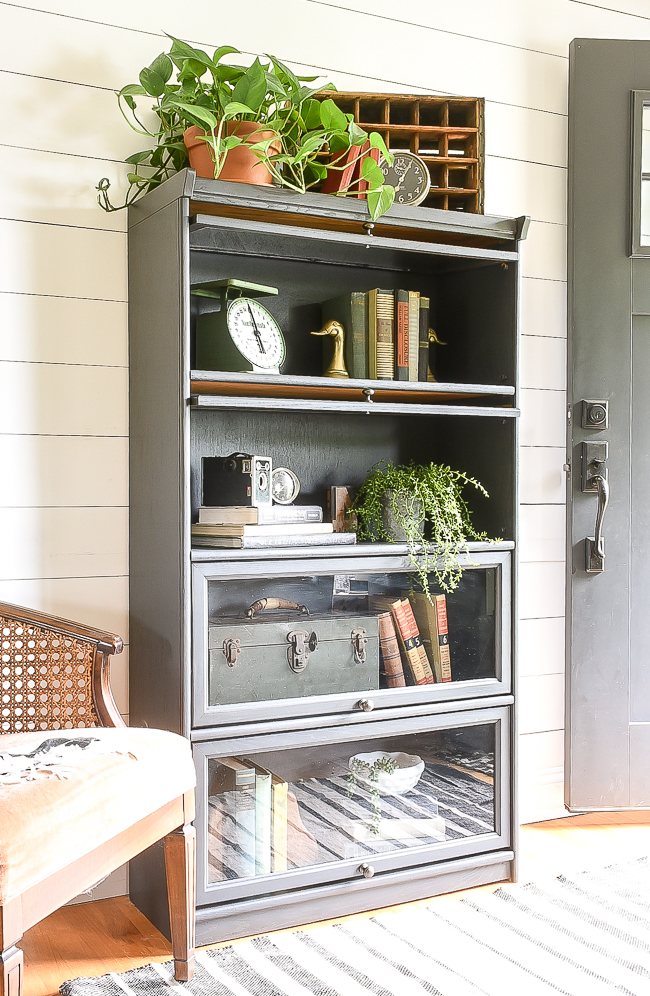This photograph, captured just inside the entrance of a home, showcases a tall, gray-toned wooden shelving unit, resembling a bookcase or cabinet, standing against a white paneled wall. The unit, approximately four to five feet tall, features a variety of intriguing items across its four shelves and more. Starting from the top, there's a lush potted plant with broad leaves cascading down, accompanied by a small, cubby-holed wooden box for messages or mail. The topmost open shelf below displays an old postal scale with a round dial flanked by a pair of golden duck head bookends securing four or five books.

The next open shelf holds an old box camera and a vintage clock resting atop a small stack of horizontally arranged books, with another plant adding a splash of green. Progressing downward, the middle enclosed section, accessible via a handle, reveals a latched trunk or safe surrounded by three books.

The bottom enclosed section, with glass doors reflecting the striped pattern of a nearby carpet, contains a mix of books and a white bowl, contributing to the eclectic display. To the right of the unit, a pink-upholstered chair with straw sides adds a nostalgic touch, despite visible wear. Further to the left, a gray door with an old-fashioned handle and locking mechanism hints at the room's vintage charm. Light streaming through a portal in the door enhances the photograph's warm, inviting atmosphere.